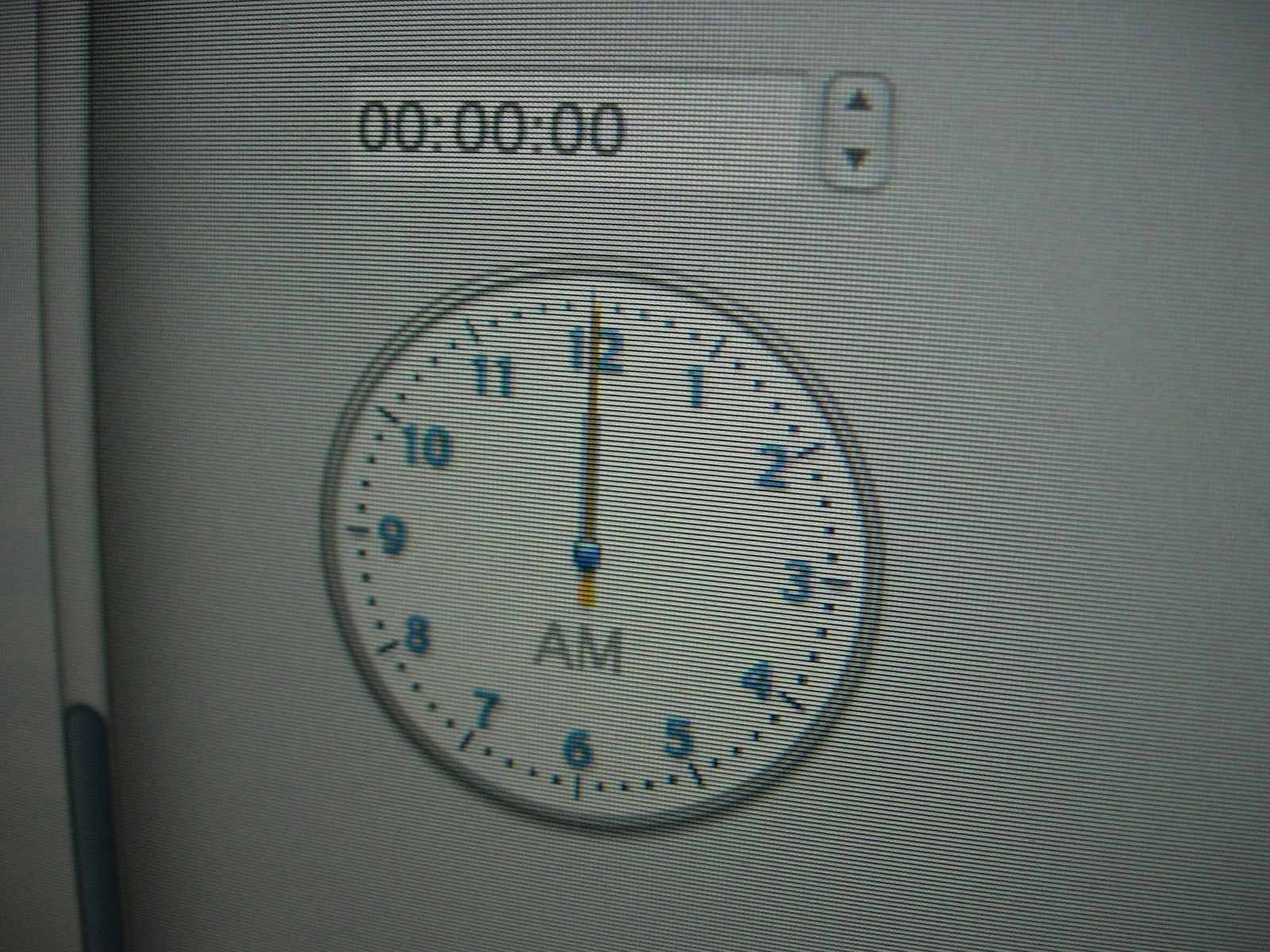A detailed photograph captures a computer screen displaying a digital clock. The image exhibits a distinct mesh-like pattern, characteristic of a photo taken directly off a screen. The clock, featuring a sleek white design, prominently displays green digits. The clock hands are positioned precisely at 12:00, indicating noon or midnight, with the descriptor "AM" situated beneath them. Above the clock, a timer is shown, set at "00:00:00." Adjacent to the timer on the right are up and down arrows, likely used for setting or adjusting the display.